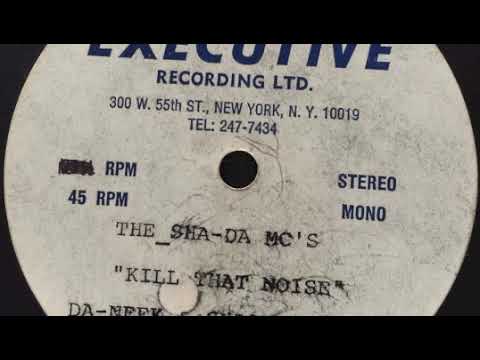This image captures a close-up view of a round vinyl record with an off-white background. The partially obscured text at the top appears to say "Executive Recording Ltd." The record is labeled "45 RPM" and includes both "stereo" and "mono" indicators, suggesting it can be played in either format. Below the top text, the address "300 West 55th Street, New York, New York 10019" is center-justified on the inner portion of the record, accompanied by the phone number "247-7434." Towards the bottom portion of the disc, underneath the center hole for the turntable spindle, the text reads "The Shah-Daz MCs" with the title "Kill That Noise." The camera cuts off the bottom and top edges of the disc, and the text is slightly angled. This vintage 45 RPM record, designed for phonograph play, showcases historical music recording details and aesthetics from a bygone era.